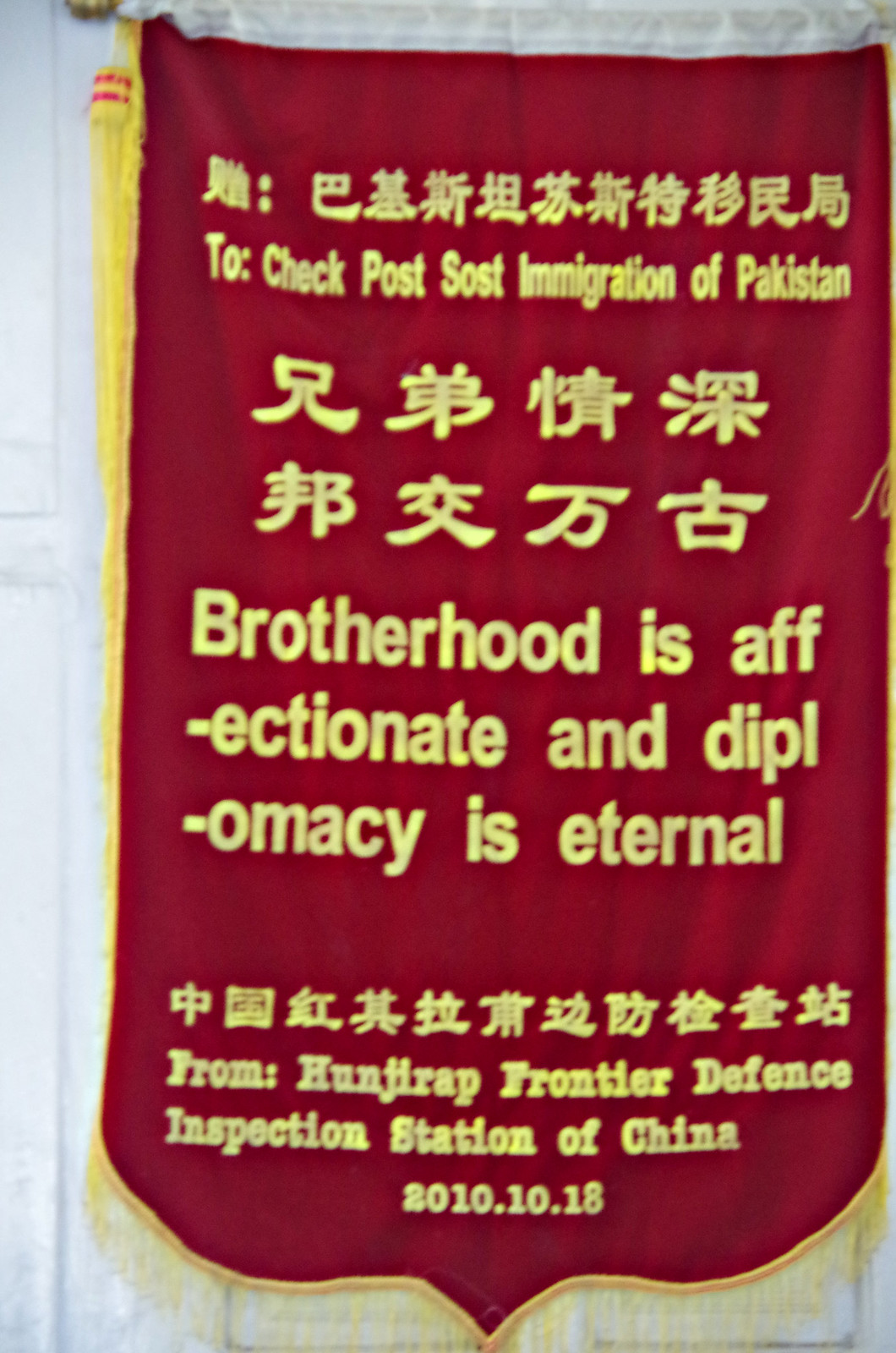The image features a large red cloth banner with yellowish-gold text written in both Chinese and English. The banner exhibits visible wrinkles and is adorned with yellow tassels on the left side, while additional tassels and a fringe appear on the bottom. The Chinese text is prominently displayed at the top, followed by the English translation "Check Post: Immigration of Pakistan". Below this, there is more Chinese text accompanied by its English counterpart stating "Brotherhood is affectionate and diplomacy is eternal". The bottom section contains another line of Chinese text and the phrase from the "Hokka Frontier Defense Inspection Station of China" along with the date "2010/10/18". The banner is centrally positioned in the image, likely hanging from the side of a building, adding to the impression of a significant and solemn proclamation.